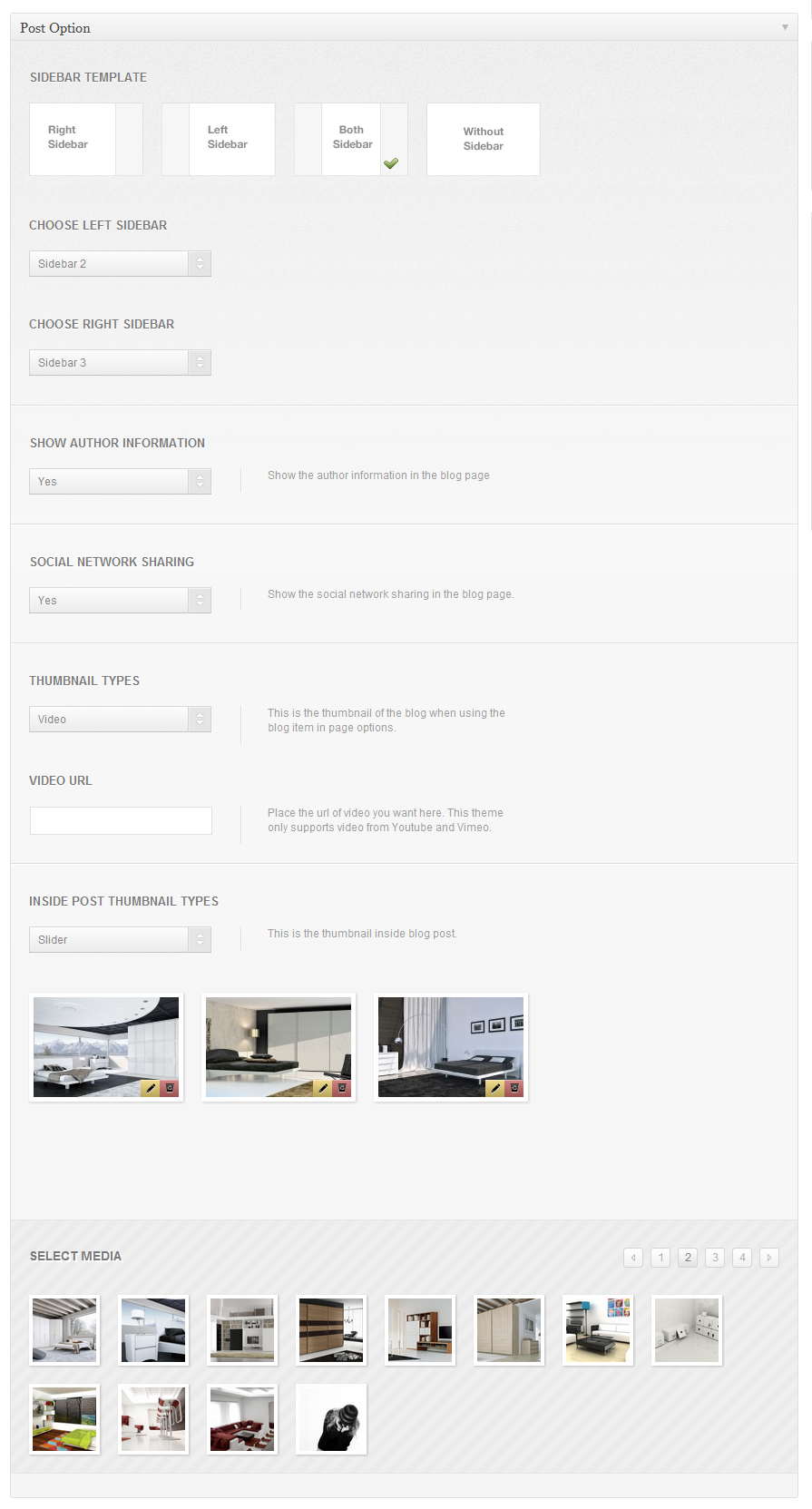The top-left corner of the image features a section labeled "Post Option" with a gray background and dark gray text. At the very top, the title "Sidebar Template" is displayed with various sidebar configuration options listed below: "Right Sidebar," "Left Sidebar," "Both Sidebar," and "Without Sidebar." The selected option, "Both Sidebar," is marked with a green tick.

Directly beneath, there is a section titled "Choose Left Sidebar," where "Sidebar 2" is selected. Another selection, "Choose Right Sidebar," indicates "Sidebar 3." Further options include toggles for showing additional information: "Show Other Information: Yes" and "Show the Social Network Sharing in the Blog Page: Yes."

In the section "Thumbnail Video," designed for displaying a blog's thumbnail when using blog items in page options, there is a placeholder for a video URL with guidance that only URLs from YouTube and Vimeo are supported. Currently, no video is entered.

The section "Inside Post Thumbnail Types" offers the option "Slider," designated for thumbnails inside blog posts. Below this, there are three images showcasing the interior of a room, predominantly white with black accents.

At the very bottom, there is a "Social Media" section displaying associated numbers ranging from 1 to 4, likely indicating different social media page settings. Additionally, there are 12 smaller images of room interiors displayed in a 2x6 grid, with 8 images on the top row and 4 on the bottom row.